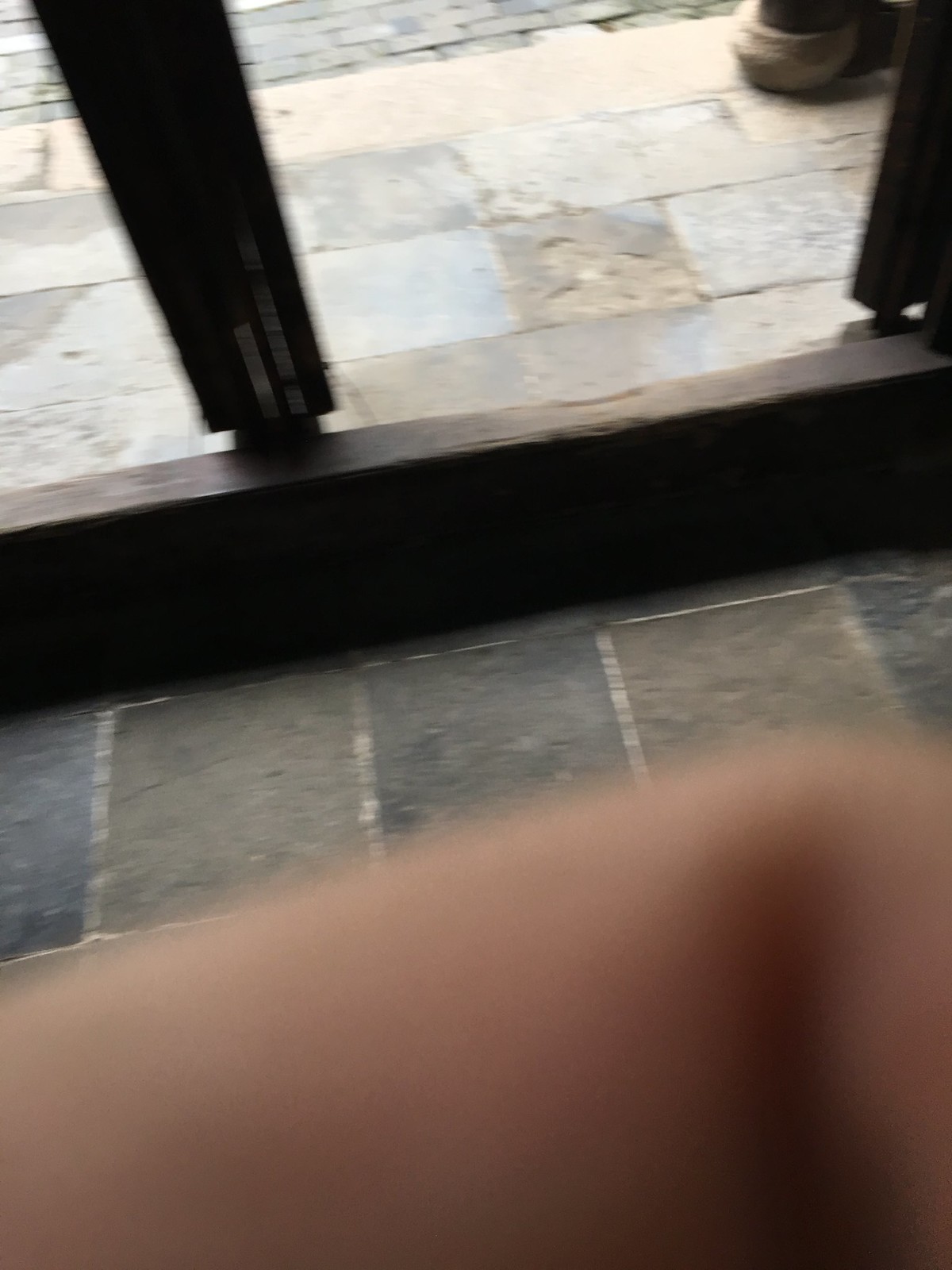The photograph captures a scene partially obscured by a human finger, which creates a blurry effect on the bottom portion of the image. Above the finger, there is a visible section of floor tiles in dark shades of gray and black. A small wooden ledge, slightly to the back, appears in the middle of the frame. This ledge features a couple of indistinct pillars, adding to the complexity of the image. In the top right corner, a tan pot is placed, contrasting with the surrounding darker elements. Despite the various elements, the image remains largely unclear due to the obstruction caused by the finger.